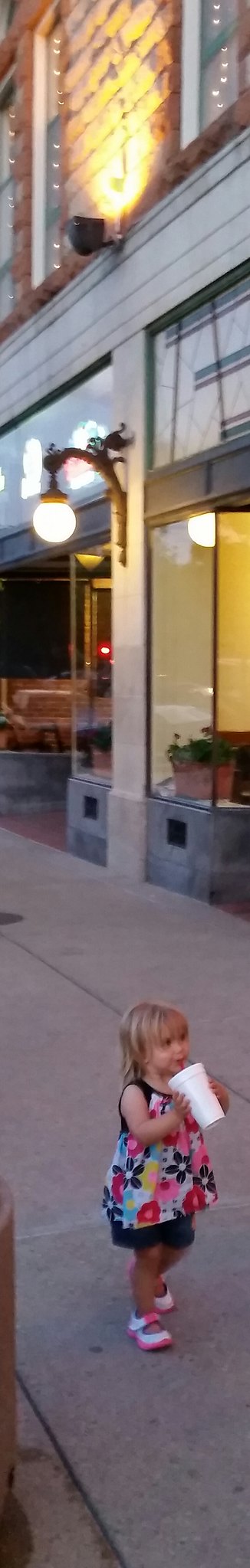In the evening light of a city sidewalk, a little caucasian girl stands dressed in a charming flower-patterned dress, complemented by blue shorts peeking from underneath. On her feet, she wears cute pink and white velcro shoes. Her shoulder-length blonde hair frames her face as she sips from a white Styrofoam cup with a red straw, her gaze directed upwards towards a figure, likely a parent, just out of the scene. The recently set sun has triggered the streetlights, casting a gentle glow on the cement slab sidewalk beneath her. Behind her, store windows adorned with various goods and stone walls create a picturesque urban backdrop. Strategically placed lights illuminate the store signs, adding to the evening's ambiance.